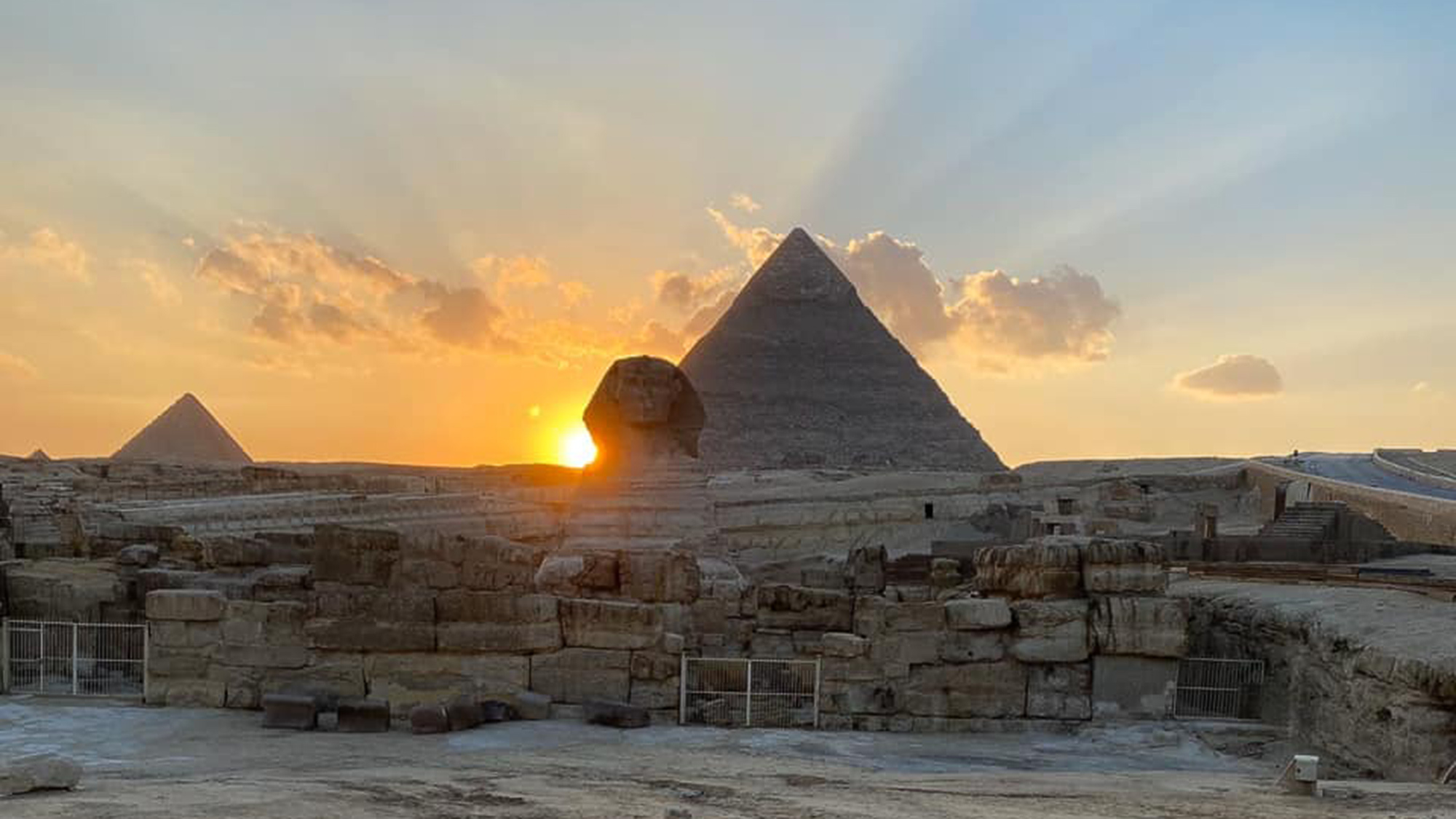This detailed photograph captures a stunning sunset over the iconic landmarks of Egypt. Featured prominently in the center is the Great Pyramid, its massive structure commanding the scene. In the foreground stands the enigmatic Sphinx, partially obscured by the intense glare of the setting sun. The sky, painted in vivid hues of orange and blue, is partly cloudy, with rays of sunlight piercing through. Below the Sphinx, several large, tan-colored stone blocks, possibly the remnants of an ancient wall, are visible, interspersed with three white metal gates. To the left on the horizon, a smaller pyramid makes its presence known. The composition of the image also includes a winding road in the distance on the far right. The absence of people adds to the timeless and majestic quality of this tableau. The serene yet dramatic lighting suggests it is more likely sunset rather than sunrise, casting a captivating glow over these ancient structures.